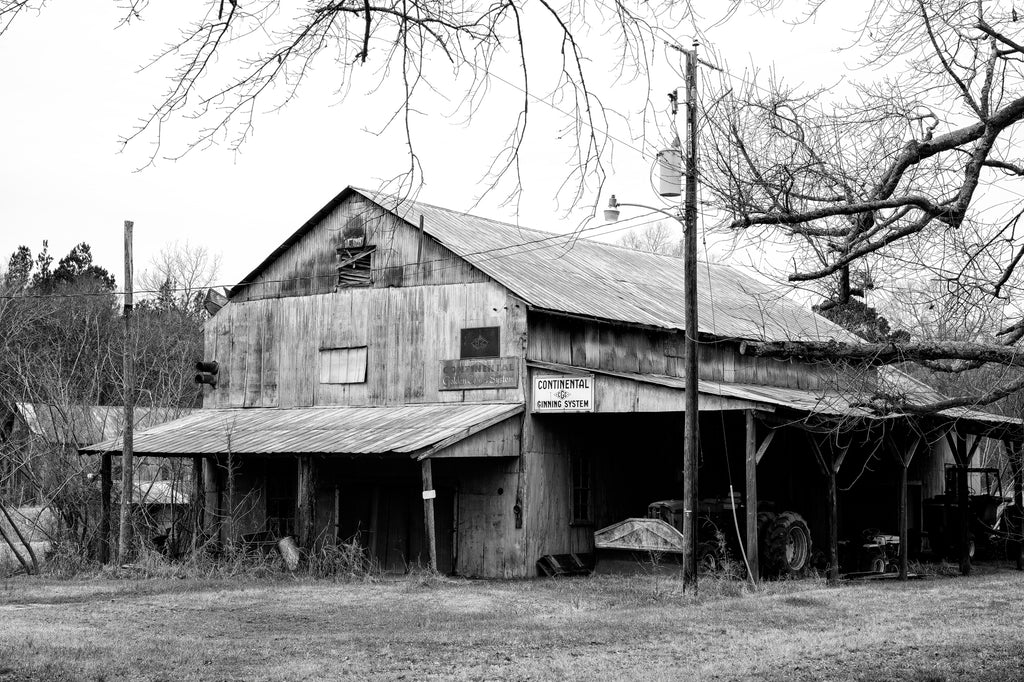This black-and-white photograph depicts an old wooden building, possibly a farmhouse or a shack, that has seen better days but isn't entirely falling apart. The structure is supported by two small poles at the front, and an awning on the side shelters two different tractors. A light pole with power lines and utility poles stands prominently in front of the building. The area surrounding the building includes numerous trees, which are bare of leaves, contributing to a desolate atmosphere. The grass in the foreground appears mostly dead, further highlighting the sense of abandonment. A weathered sign on the building reads "continental" or possibly something related to "system," though it is difficult to decipher due to age and wear.